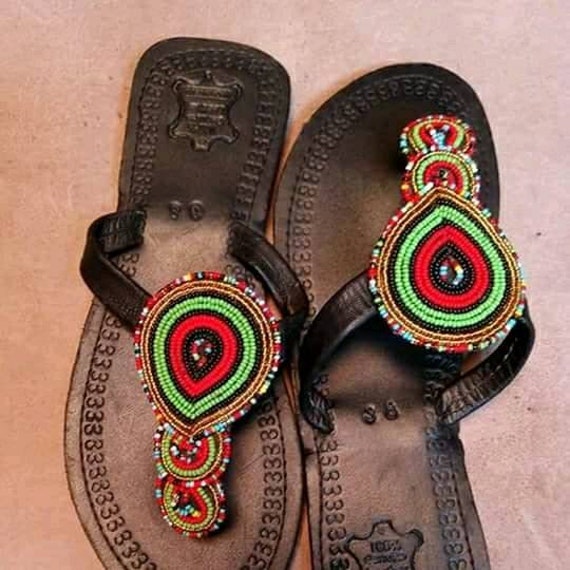This image captures a pair of new dark brown leather sandals set against a terracotta-colored tile floor. The muted, slightly grainy quality of the photograph suggests it could be from an older slide or taken with studio lighting that has faded over time. The sandals are positioned side by side but with their toes pointing in opposite directions — the left sandal is front and center, pointing downward, while the right sandal is to the right and pointing upward.

The sandals feature intricate details, particularly on the upper strap and thong area. Elaborate beadwork in a paisley pattern decorates the top, comprising bands of black, lime green, and red beads. Additionally, there are multicolored bands forming light, circular patterns, including two smaller near-circles and a larger teardrop-shaped design. A small jewel is embedded in the bead arrangement, and this pattern repeats three times along the thong.

An etching resembling the number '3' loops around the sole, extending through the heel. Inside each heel, there is a logo of the sandal's maker. The overall color palette of the beads and embroidery contrasts with the subdued brown leather, adding a colorful and detailed focal point to these distinctive sandals.